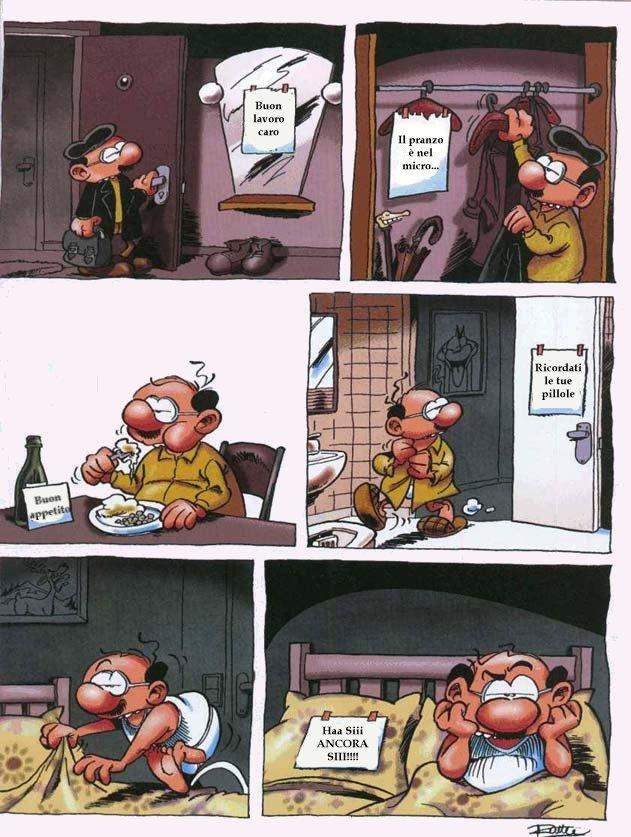This detailed comic strip in a foreign language comprises six panels arranged in two columns and three rows. It features a short, middle-aged man with male pattern baldness, a giant nose, glasses, and a hat. He appears to be arriving home and going through his nightly routine. 

In the first panel, we see him entering his house or apartment, noticing a note on the mirror that reads "Buon Lavoro Caro." 
In the second panel, he removes his jacket and hangs it up in the closet, where another note, "El Prazo, El Nel Micro," is attached.
The third panel shows him at the dining table, eating what looks like mashed potatoes. A note on the table says, "Buon Appetit."

Moving to the fourth panel, he walks towards the bathroom, where another note is posted on the door, reading "Riccardo Attu Pillolo."
In the fifth panel, he is getting into bed, dressed in white pajamas, but this scene does not have any text.
Finally, in the sixth panel, the man is lying in bed with his hands on his cheeks, looking disgruntled. A note on the pillow next to him is in capital letters, saying "Hassel and Cora Sitt."

The bottom right corner of the comic strip contains the artist's autograph, which is slightly unclear but appears to read "Rattay" or "Portay."